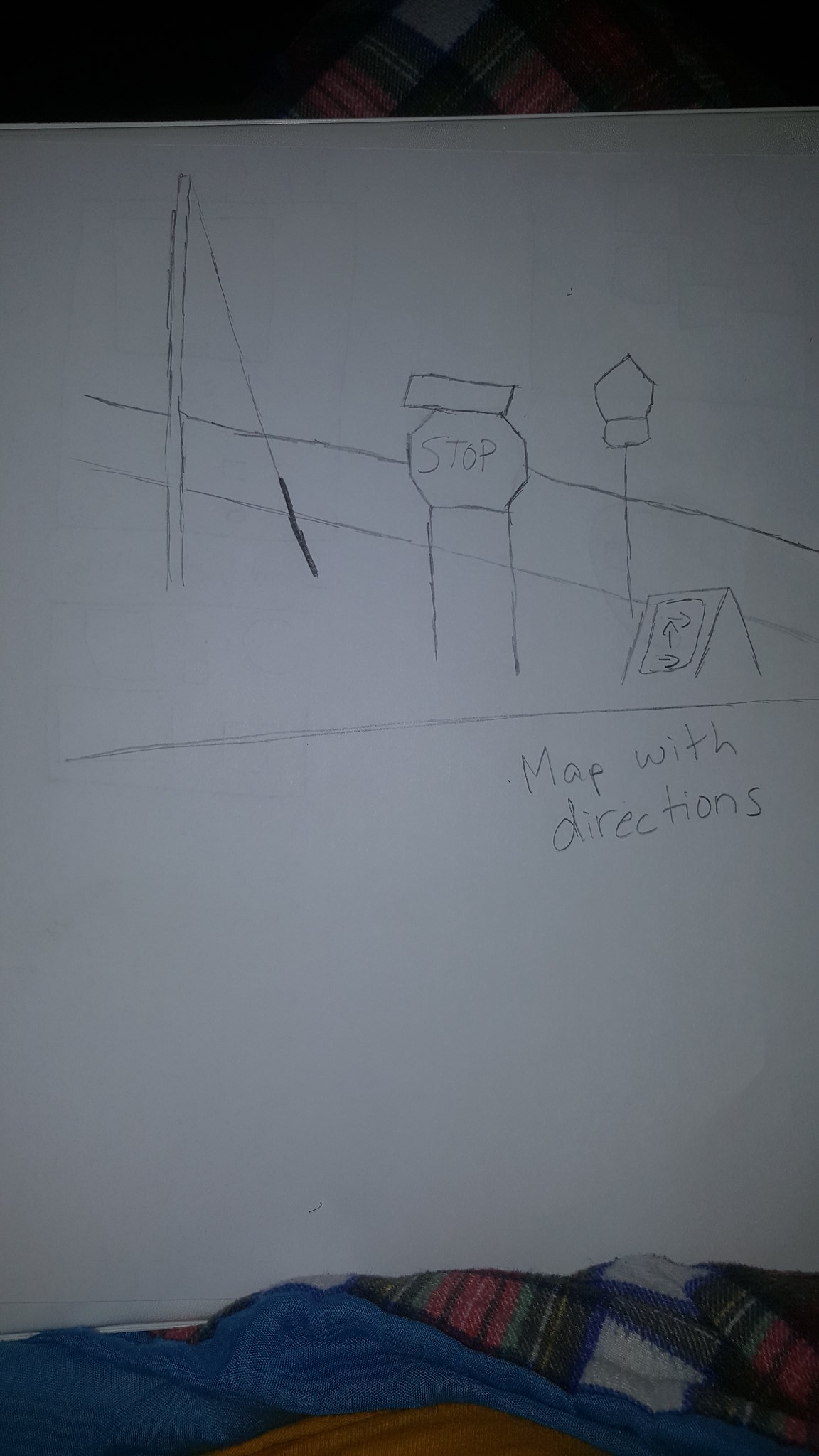This photograph captures a rudimentary pencil drawing, likely created by a child or someone inexperienced in drawing. The sketch appears on a white surface, possibly paper or a whiteboard, and is placed atop a bed with several crumpled blankets in the background. These blankets are multicolored, with shades of blue, green, and red.

The focal point of the drawing is a stop sign, recognizable by its characteristic octagonal shape and the word "STOP" written inside. Above the stop sign is a rectangular shape, supported by two simple vertical lines representing posts, indicative of an elementary perspective attempt.

In the background of the drawing, two horizontal lines mimic the appearance of a fence. Additionally, there is a depiction of another street sign and a caution sign like those used to indicate a wet floor. This caution sign displays arrows pointing right, up, and right again, with the words "MAP WITH DIRECTIONS" inscribed on the surface. The entire composition is rendered in pencil, distinguishing it as a straightforward line drawing. The dim upper part of the background makes it hard to discern further details.